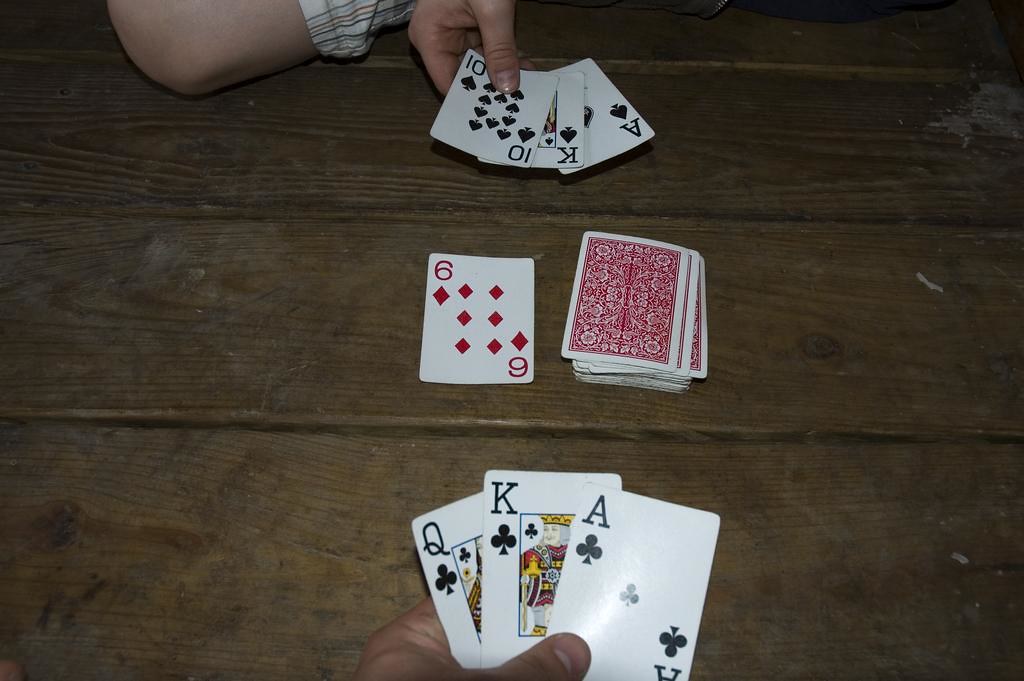This color photograph captures an overhead view of a rustic, seemingly worn wooden floor where a group of people are engaged in a game of cards. The surface of the floor—covered in scratches and marks—suggests it is not polished and has seen significant use. 

At the top of the image, there is a bit of ambiguity; what looks like either a knee or an elbow protrudes into the frame, further suggesting that the individuals are seated on the floor. A right hand extends from the top center, laying down a ten of spades, a king of spades, and an ace of spades—revealing a decisive move in the game.

In the middle of the floor, a neatly stacked deck of cards lies face down, marked by a red and white pattern with a white border. Beside this deck, a six of diamonds lies face up, hinting at the progression of the game.

Towards the bottom center of the photograph, another participant's left hand is visible, seemingly mid-play. This hand, which appears masculine, holds a queen of clubs, a king of clubs, and an ace of clubs, reflecting a similarly strong stance in the game. These cards catch some light, highlighting their glossy surface.

Overall, the image effectively captures the informal and relaxed atmosphere of a friendly card game, played on a well-worn wooden floor.